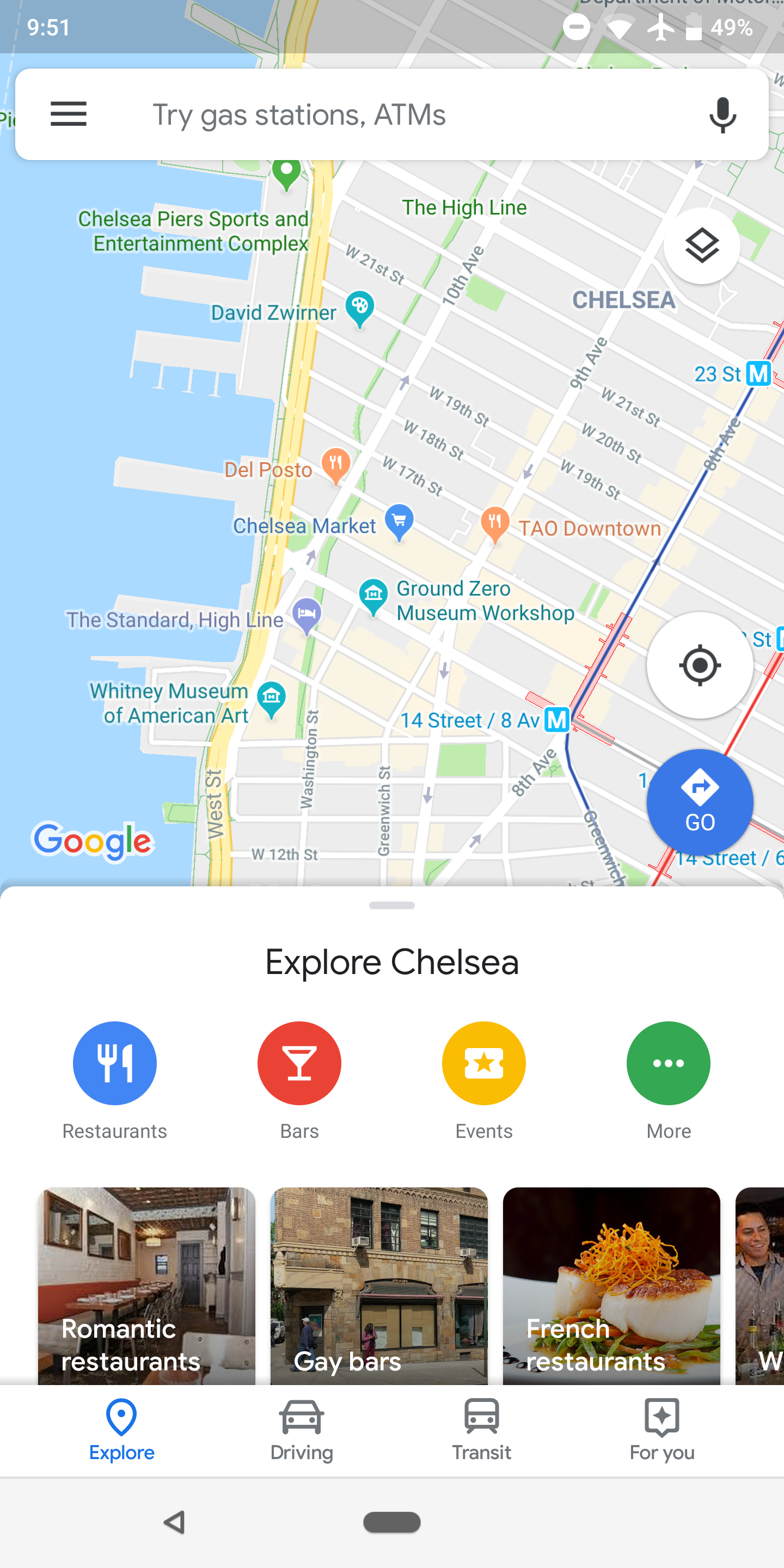A detailed screenshot from a cell phone displaying a Google Maps page taken at 9:51 AM with the device in airplane mode and the battery at 49%. The map focuses on downtown New York City, specifically near the Chelsea area, displaying notable landmarks such as the Ground Zero Museum, Chelsea, 14th Street, and Piers. At the top of the screen, there is a search bar accompanied by a microphone icon and a menu option. Within the search bar, suggested search options like "gas stations," "ATMs," and "restaurants" are visible. Below the map, a section titled "Explore Chelsea" presents predefined categories including "restaurants," "bars," "events," and more. Thumbnail images and topics like "romantic bars," "gay bars," and "French restaurants" are showcased. At the bottom of the screen, there are icons for "explore," "dining," "transit," and a personalized "for you" section.